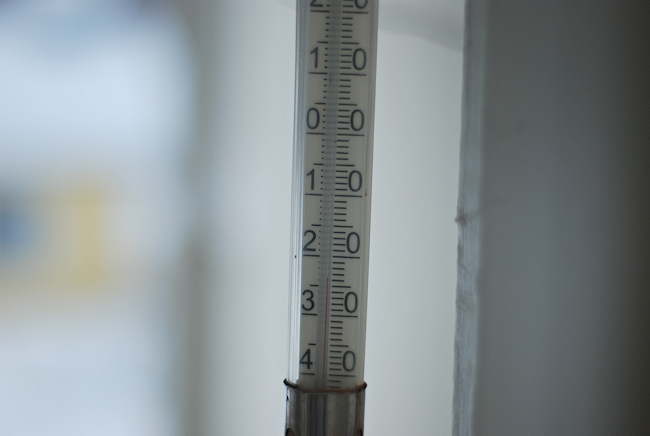The image prominently features a white thermometer, extending vertically from the top to the bottom of the frame. The thermometer's central red mercury line indicates a temperature just above the 3.5 mark on the scale. On the left side of the thermometer, the scale ascends from 4 at the bottom, climbing up through 3, 2, 1, 0, and continuing positively with 1 and 2. The right side of the thermometer displays a series of zeros. Measurement lines are clearly visible on both sides of the scale.

The thermometer is encased in a plastic base situated near the bottom of the image. The background is intentionally blurred, showcasing the depth of field effect. A piece of a white wall or door is visible entering from the right side of the frame, casting a subtle shadow, adding contrast. The setting seems to be a white hallway with a doorway on the left. Inside the adjacent room, indistinct blue and yellow shapes can be seen, further contributing to the overall blurred ambiance of the background.